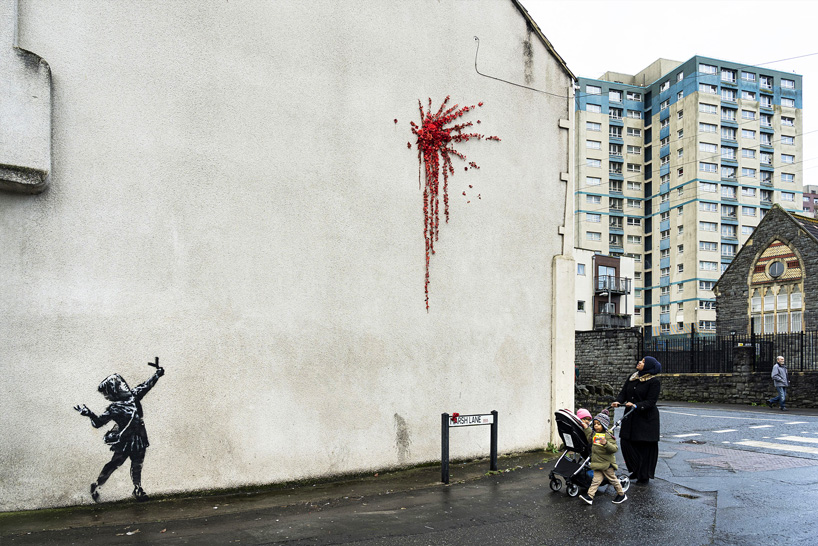The image depicts a rainy, overcast street corner in a European town, dominated by the side of a large, white building. The building features an eye-catching mural: a small Victorian-era boy, illustrated in black and white, holding a slingshot. The arc of the slingshot leads to a vivid red explosion evocative of splattered petals or flowers. Below the mural, a woman dressed in black robes and a hood, likely the children's mother, pushes a stroller. One child, wearing a pink cap, sits in the stroller, while the other, in a grayish-brown cap, walks beside her. The scene is enriched by the backdrop of diverse architectural styles, including blue-and-white multi-story buildings and some brick structures, adding depth and context to the urban mural setting. A passerby glances at the mural, adding a touch of everyday life to this evocative street tableau.